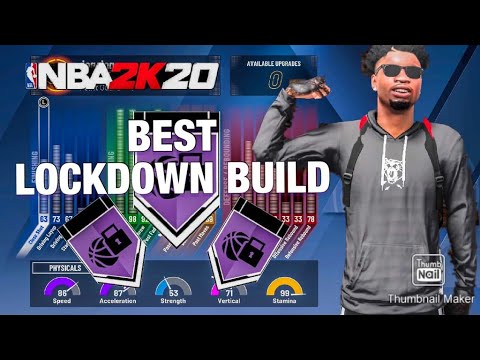Here is a polished and detailed caption based on the provided description:

---

This web page for NBA 2K20 prominently features the NBA logo on the left side. On the right side, it displays the term "Available," followed by a zero. The central image showcases an African American individual wearing dark sunglasses and a gray hooded sweatshirt with a single front pocket. The person, who appears thin and is carrying a backpack, stands confidently, embodying the concept of the "Best Lockdown Build." Accompanied by two tags featuring black silhouette images of basketballs and locks, the page further emphasizes the character's defensive prowess. Below this, the physical attributes are listed, including Speed, Acceleration, Strength, Vertical, and Stamina, allowing players to gauge their abilities. The page also mentions "Thumbnail Maker," likely referring to the tool used to create the thumbnail, along with a nod to NBA2K20.

---